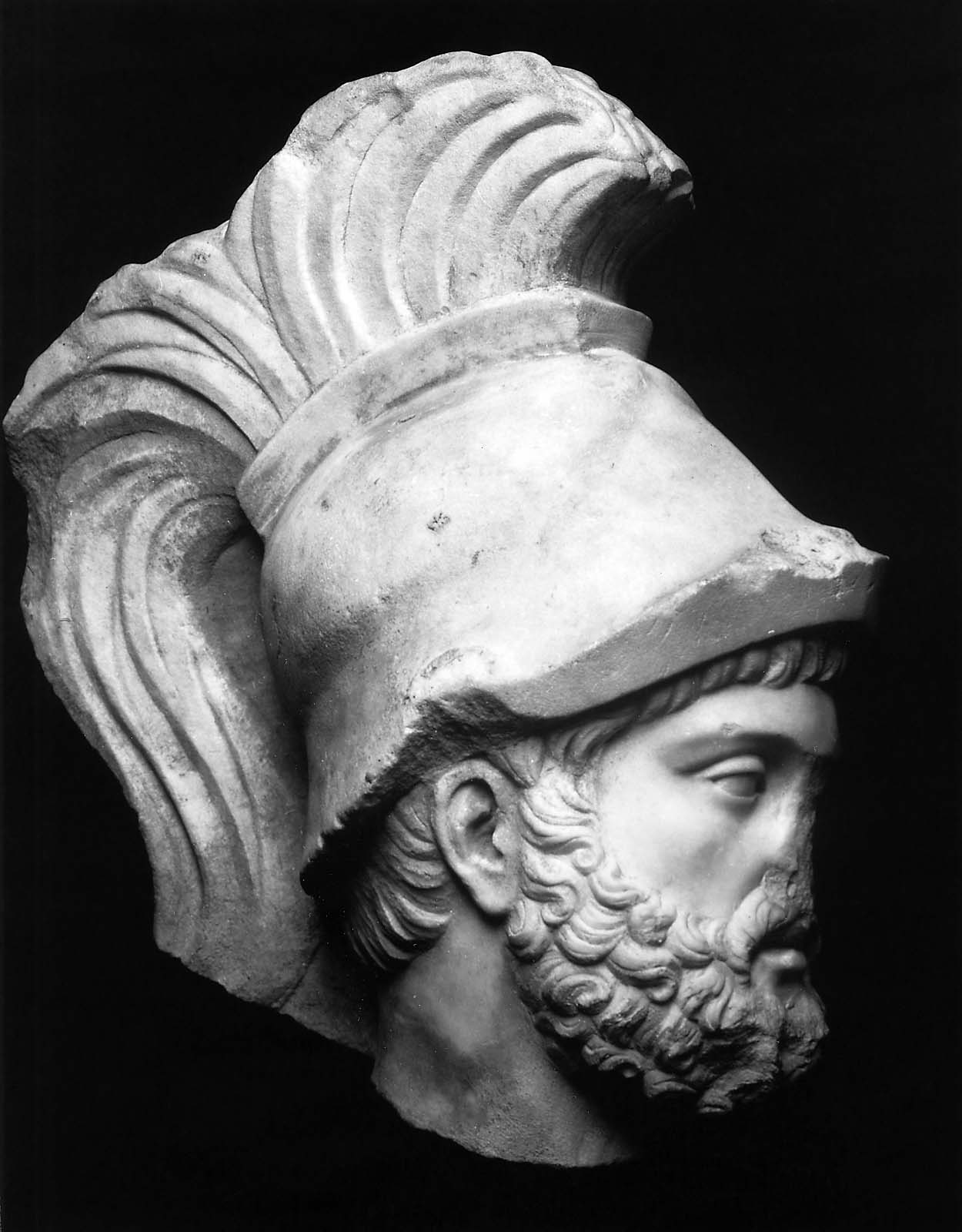The image depicts a marble statue head of a Greek god, viewed from the side against a black background. This head appears to be broken off from a larger statue and captures meticulous details from the neck upwards. The Greek god has short, curly hair barely visible under an elaborate helmet. The helmet, tall and adorned with a plume that stretches both forward and backward, shows signs of damage with chips and broken segments. The deity sports a thick, long, and curly beard, along with a mustache, although the nose and parts of the mustache are broken. The statue's ear is visible, and the mouth appears slightly open, revealing the worn beauty of this ancient artifact.